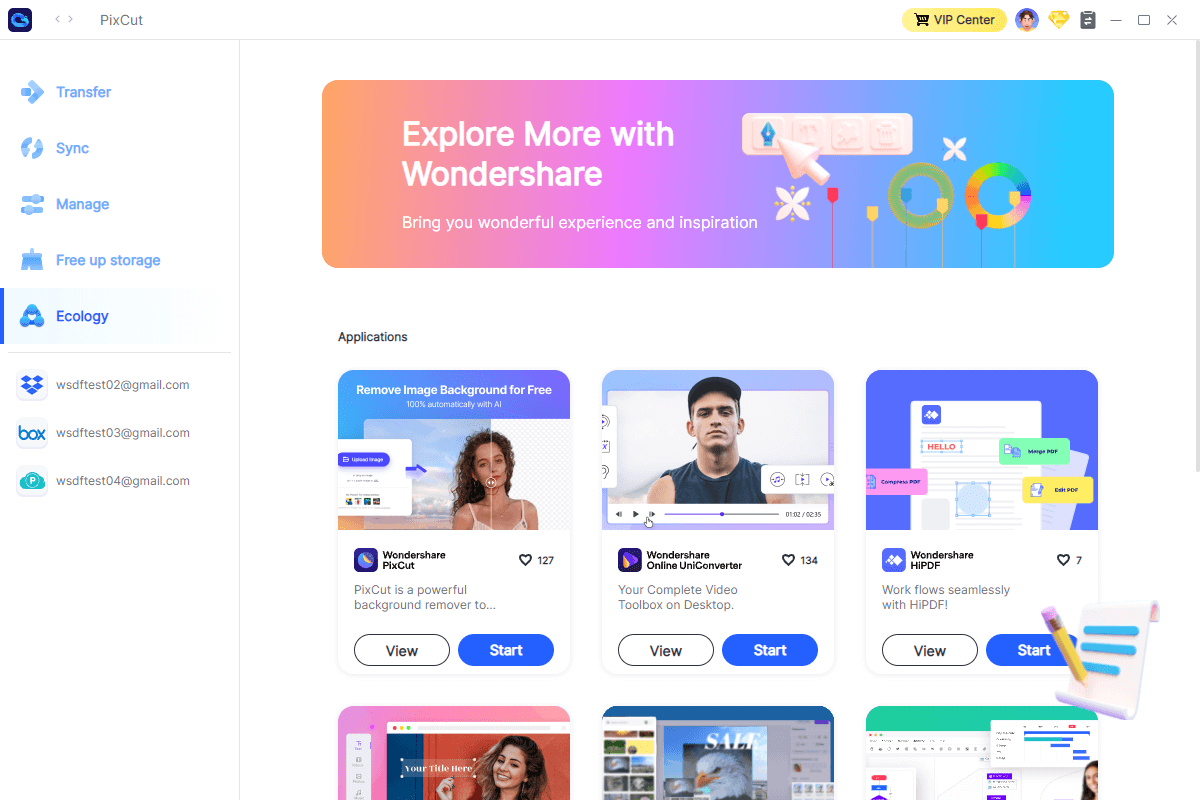This image, sourced from a website named PIXCUT (spelled P-I-X-C-U-T), displays a user interface against a white background. Prominently positioned in the upper left corner is a blue symbol. On the opposite end, the upper right corner features a shopping cart icon and a VIP Center button, accompanied by a user icon and additional icons.

Running down the left side of the screen, there are blue labels labeled 'transfer,' 'sync,' 'manage,' 'free up storage,' and 'ecology.' Below these labels, three email notifications are visible.

On the right side of the image, the top portion showcases a colorful block comprised of pink, peach, lavender, and blue hues, adorned with rainbow-colored rings, a white arrow, and a green ring. This section contains the text "Explore more with Wondershare." 

Beneath this header, within the applications section, six tiles are displayed. The first three tiles are fully visible, while the bottom three are partially cut off. Each tile includes both a 'view' and a 'start' button beneath it.